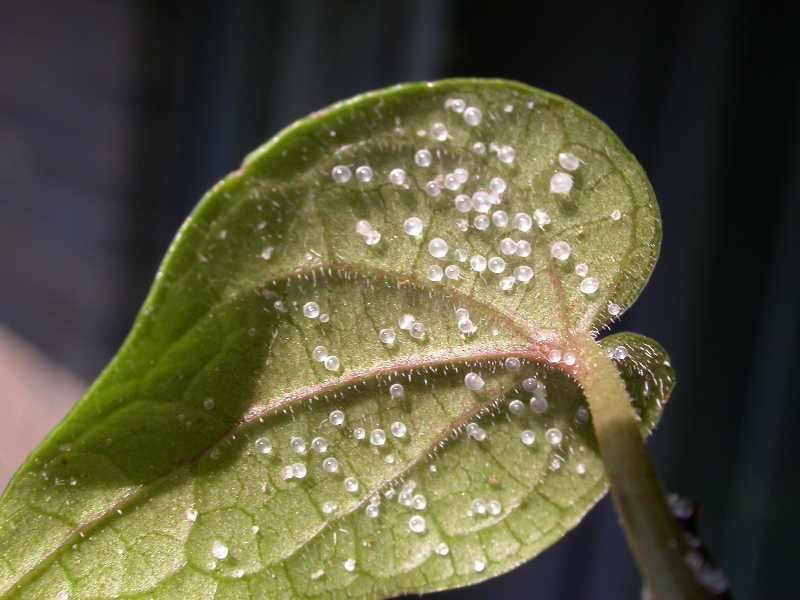The image shows a highly detailed, close-up view of the underside of a green leaf, with a distinct focus on its intricate vein structure which is tan to red in color. The leaf is populated with numerous small, white dots that are possibly eggs, alongside clear, bubble-like water droplets scattered across the surface. The background is an almost black, shadowy blur which accentuates the darker and lighter blackish-blue tones, making the leaf stand out prominently. The stem of the leaf extends diagonally towards the bottom right corner, providing additional context within the image's overall composition. The photo is extremely clear, capturing the fine details—including the tiny hairs along the veins—under natural lighting, and features no additional elements such as words or numbers.